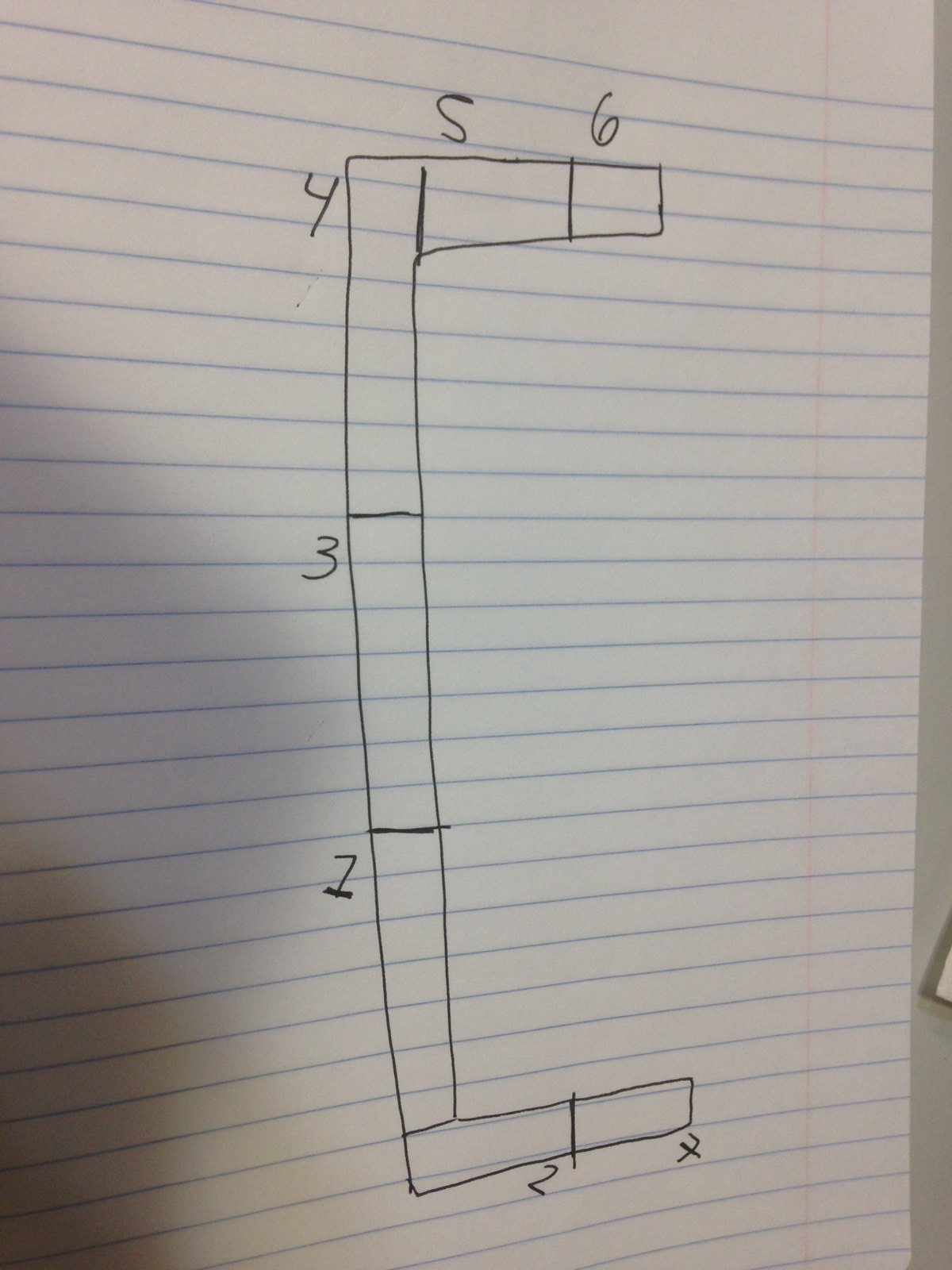A photograph features a sheet of college-ruled lined paper. The paper has faint blue horizontal lines and a vertical red margin line on the left side, indicative of standard notebook paper. This particular sheet appears to be the backside, inferred from its translucent quality. On the paper, a geometric sketch is prominently visible. The drawing appears to be an irregular block-like shape, divided into several sections. Various numbers label these sections: "5" and "6" are written on the top, while the sides are marked with "4," "3," and "1." The bottom sections bear the numbers "2" and "7." The intricacy and layout of the sketch suggest that it might be part of a mathematical problem, possibly to determine the perimeter or volume of the shape. The detailed annotations and structured nature of the drawing indicate an effort to solve or visually represent a mathematical exercise.